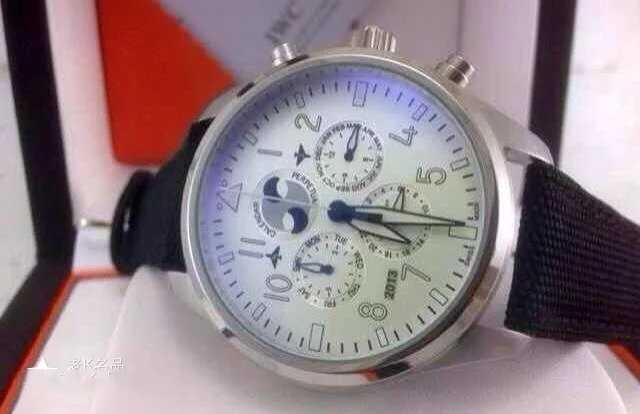This detailed image depicts a close-up of a sophisticated wristwatch, displayed on its side within a square case against a red and gray background. The watch features a black fabric band and a silver-colored stainless steel bezel. The main dial is complex, divided into four sections, including a large analog timekeeping dial and three smaller stopwatch functions. The hour hand is a long, skinny diamond shape, while the minute hand is a shorter diamond shape; the second hand is a thin white line pointing close to the 12 o'clock mark. Notably, the numbers on the watch face are white with black outlines, and instead of numerals at 12, 3, 6, and 9, there are distinctive markers—rectangles, except the 12, which is a triangle. The subdials include indicators for the month, weekdays, and calendar days. Additionally, the lower left corner of the watch shows the year 2013, suggesting the photo's age. The timepiece is elegantly crafted, combining functionality and aesthetics, complete with three side buttons for stopwatch functions and time setting.